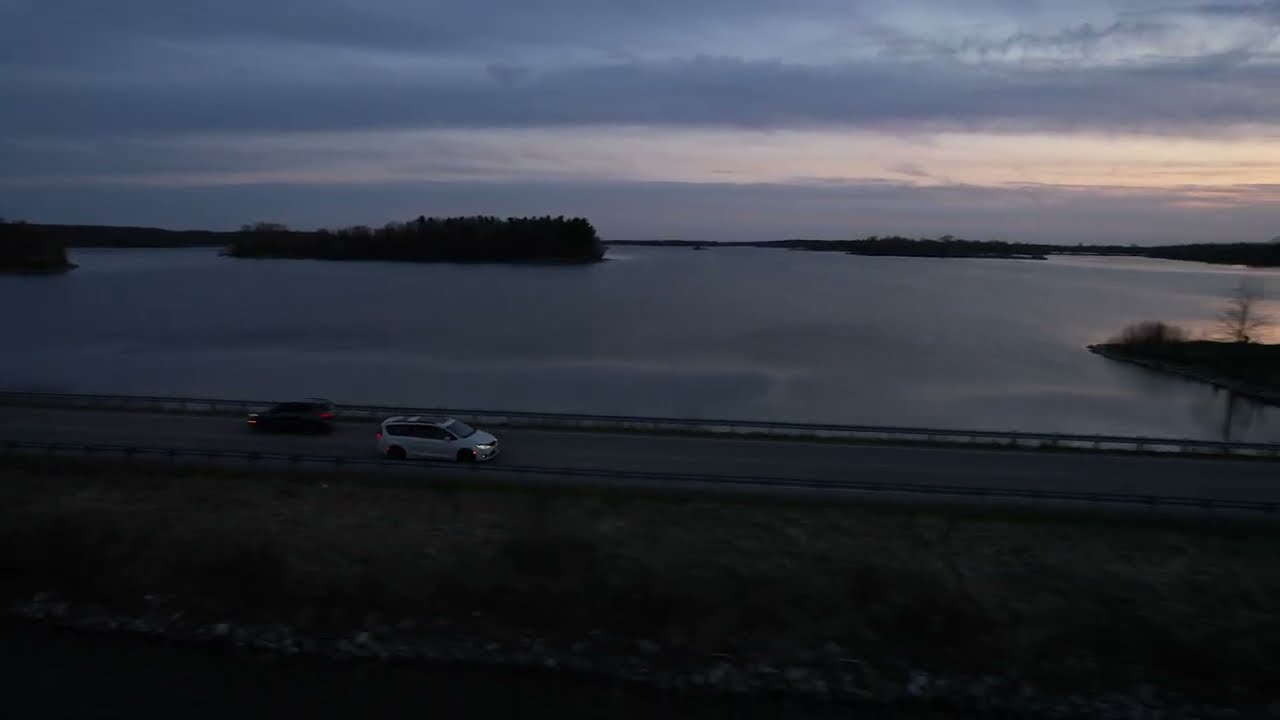In this evocative photograph taken at sunset, a serene lake stretches out to the horizon, accented by a glowing afterglow of the setting sun on the right. The calm waters mirror the fading light, while several islands dot the expanse, the nearest island crowned with a barren tree. In the foreground, a two-lane roadway hugs the shore, bordered by safety railings. A white SUV with headlights on travels to the right, while a darker vehicle moves in the opposite direction, its lights indeterminate. A dark boat can be seen on the tranquil waters in the distance. There are no lights or buildings in the image, and the sparse, leafless tree suggests a winter setting. The landscape, framed by gentle hills, captures a moment of quiet beauty in shades of twilight gray.